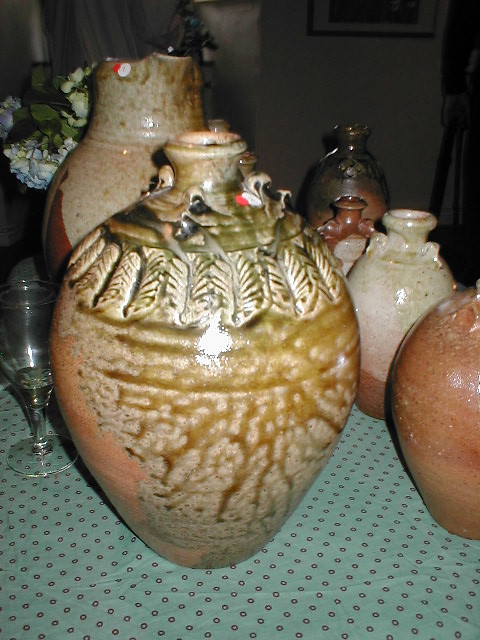This photograph captures an assortment of handcrafted clay vases displayed on a table adorned with a seafoam green tablecloth dotted with rows of evenly spaced black circles. Dominating the table are two prominent vases, with narrow openings designed to hold items, possibly even water. In front of these, closer to the table's edge, stand three medium-sized vases and a smaller, rosy-peach colored one. The vases exhibit a palette of earthy tones, including brownish salmon, rusty red, golden, and light reddish hues. The largest and second-largest vases feature intricate leaf imprints around their necks with beige leaves veined in green, and a green-to-brown gradient dripping down their bodies. Also on the table, there is a crystal clear wine glass adding a touch of elegance to the arrangement. In the background, a few plastic blue and white flowers drape down, providing a hint of decoration behind the artistic pottery display.